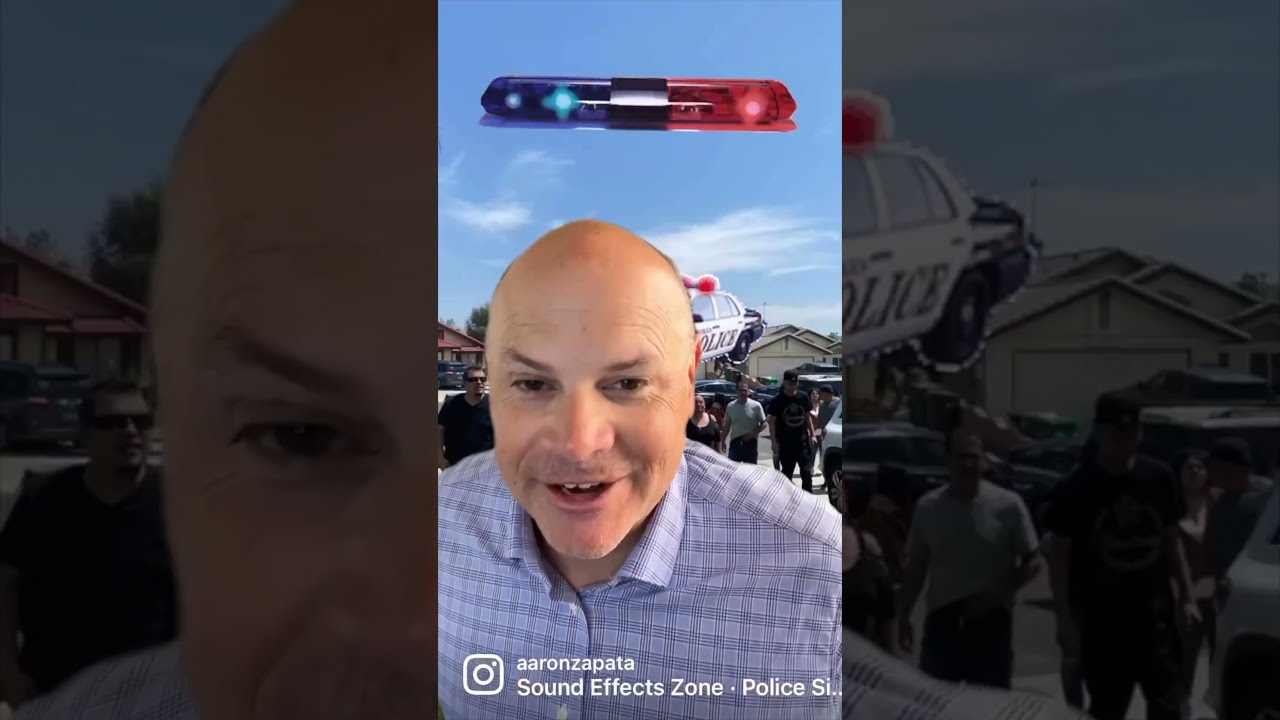The image features a bald Caucasian man, likely older, positioned towards the bottom middle of the frame. He is leaning forward with his mouth open, revealing his top teeth, and has a faint mustache and beard. He is dressed in a blue plaid button-up collared shirt. The background showcases a scene with people, cars, and houses lining a subdivision. Floating in the sky behind him is an edited police car and a light bar, with the police lights displayed as blue on the left and red on the right. There are borders on both sides of the image, containing close-up views of elements from the main picture. At the bottom left corner, the Instagram logo appears next to the name "Aaron Zapata" and the text "sound effects zone police SI" is written underneath.